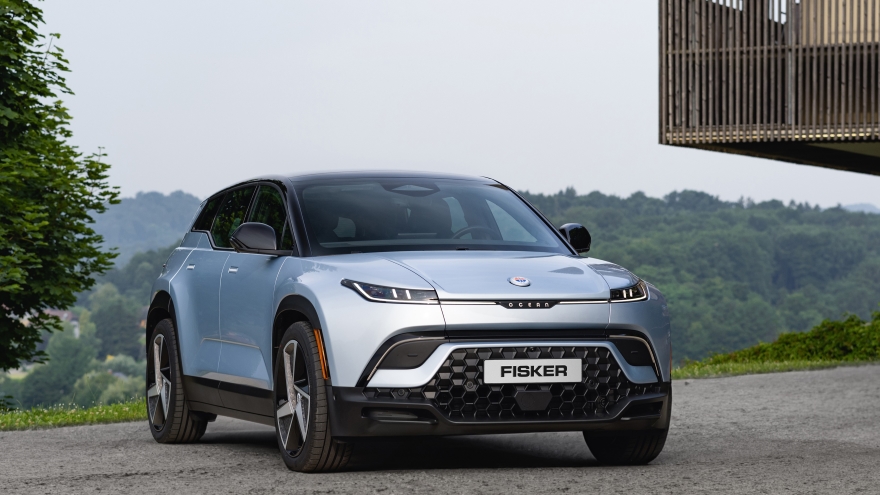The image showcases a greyish blue Fisker SUV parked on an asphalt pavement or concrete surface, with the word "FISKER" prominently displayed on the front grille and smaller lettering, possibly "OCEAN" or "delta," near the front hood. The contemporary car features a sleek design with orange detailing on the lights. The background, though somewhat out of focus, reveals a scenic setting with tree-covered hills and a lush forest visible in the distance. There is a tree or bush on the left side of the image, and a small patch of grass with tiny flowers adjacent to the car. Additionally, a wooden structure, likely a balcony or deck, is partly visible in the upper right corner, extending out from a building, suggesting the car is parked in front of a hillside home. The overall scenery behind the vehicle is picturesque, emphasizing the natural beauty of the location.